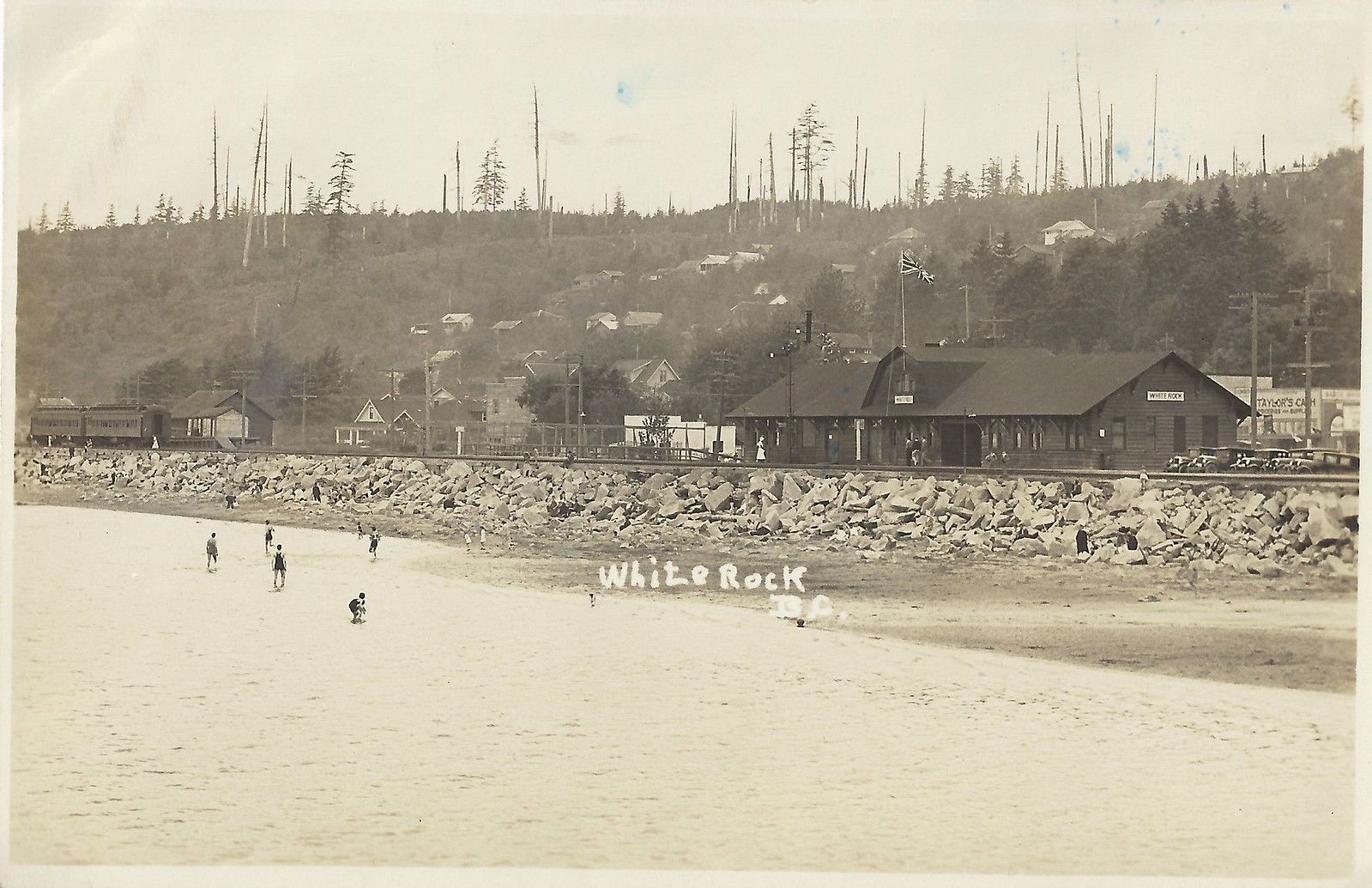This is an old black-and-white photograph capturing a tranquil lakeside scene with a bustling beach. The lake occupies the left side of the image, shallow in depth, as multiple people stand in ankle-deep water. The beach, a narrow sandy strip, seamlessly transitions into a barrier of large boulders that support an elevated train track. 

Central to the composition is a white marker with the inscription "White Rock BA." To the right, set above the rocky barrier, is a single-story train station, characterized by its dark sloped roof and prominently displayed large British flag on a flagpole. Adjacent to the station are a few additional wooden buildings, which likely serve as homes or auxiliary structures.

The background features gently sloping hills dotted with sparse, leafless trees and tall, thin trunks. A train is visible, having just departed the station, its rear end extending off the left edge of the frame. This evocative image with its horizontal orientation and detailed landscape illustrates a moment in a serene yet active lakeside community.